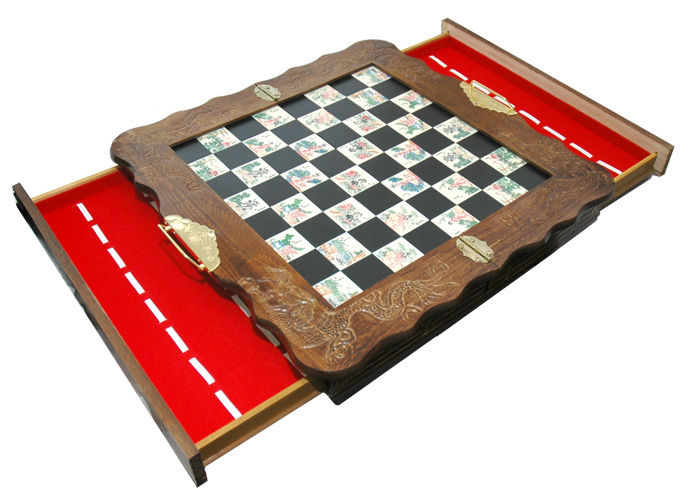This image showcases an intricately designed game board set against a stark white backdrop. The board itself has a folding hinge, allowing it to be easily stored or transported. Its edges are adorned with wooden trim, featuring detailed etchings of dragons at each corner, adding an element of artistic flair. The playing surface resembles a classic checkerboard, with alternating black and white squares. Each white square contains unique illustrations, which may serve a specific purpose in the gameplay. Additionally, the game board features practical functionality, with drawers on both sides. These drawers have striking red interiors lined with white strips, likely designed to secure the game pieces in place when not in use.